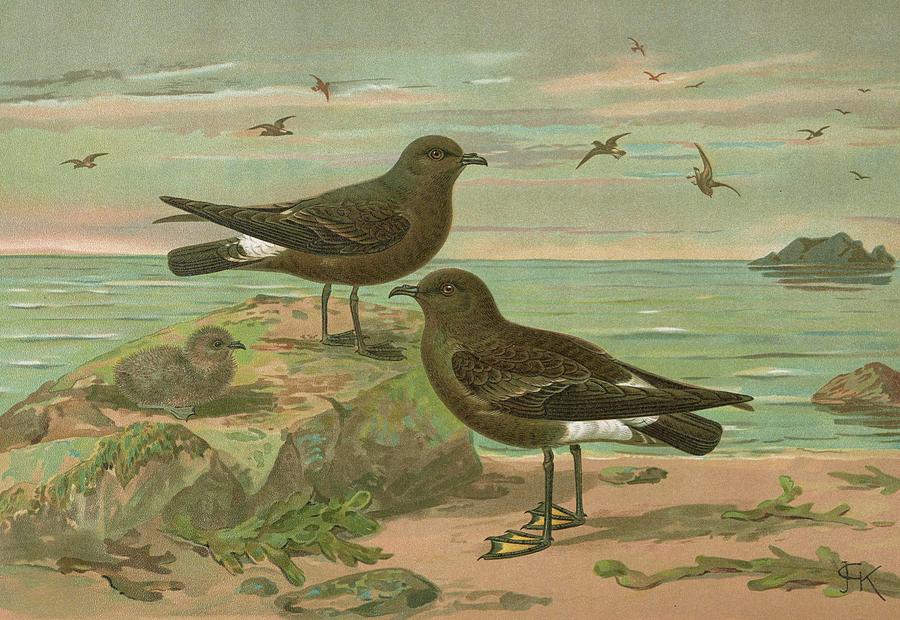This is a detailed, illustrated painting of a serene ocean scene at the beach, rendered in muted, dark colors giving it a grainy texture. The painting features several birds, which may be seagulls or another type of sea bird, highlighted in various poses. A large, algae-covered rock sits prominently in the foreground, showcasing green moss and earthy brown markings. Perched atop this rock is an adult bird with a dark brown body and black beak, facing to the right, accompanied by a fluffy, light tan baby bird. On the sandy beach in front of the rock stands another adult bird facing to the left, sharing similar brownish hues with darker wings and black beak, along with some characteristic white marking near the tails.

The sand is depicted with strewn seaweed, random foliage, and scattered pebbles, adding to the beach's natural detail. Extending towards the background, the tranquil teal ocean displays subtle white caps and various shades of blues and greens, accentuating the calmness of the scene. Among the waves sit additional rocks, including one larger formation resembling a small island. Above, the sky occupies about a third of the painting, showing a softer palette of gray, peach, blue, and pink hues that differentiate it from the sea. The sky also features several birds soaring in the distance, completing this picturesque and richly detailed oceanic illustration.